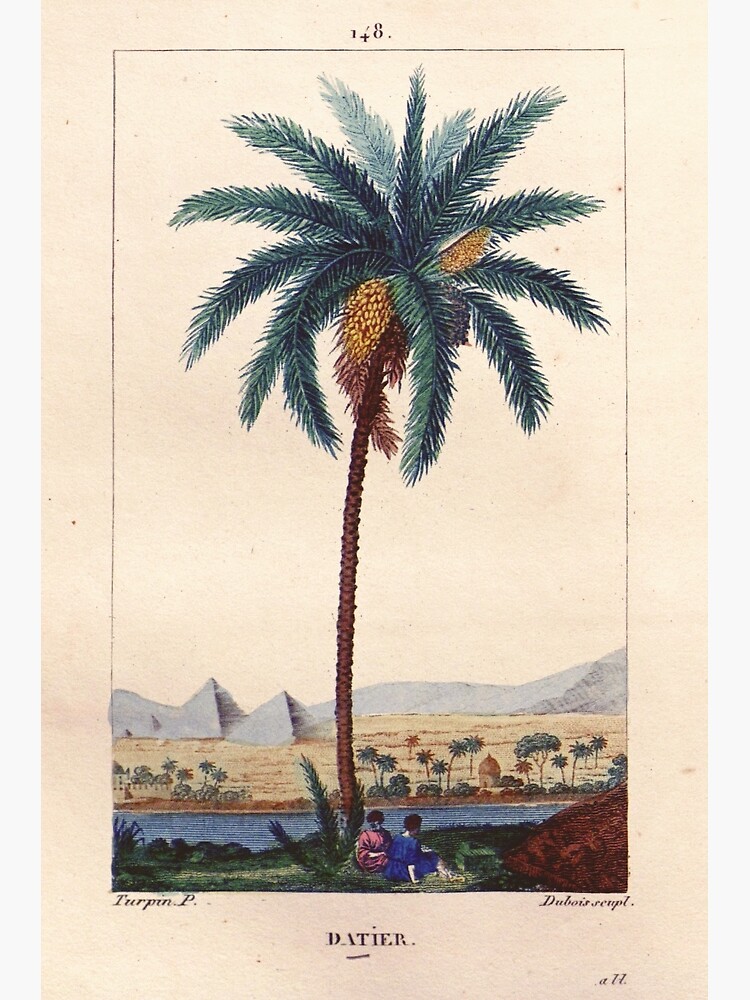The image appears to be a hand-drawn, painted illustration, possibly from a card or book, featuring a central palm tree with green leaves extending in various directions, and a long, curving brown trunk. The background is cream-colored with a thin black outline. The primary focus is the palm tree, which has what seems to be bananas or brown fruits hanging from the center. The foreground shows a green oasis with two figures sitting beneath the tree—one wearing blue, the other pink. In the background, a blue river flows across, with additional small trees lining its banks. Beyond the river, the landscape transitions into a sandy desert displaying pyramids, hills, and a few buildings.

The top of the image is white or off-white, while the bottom features a light brown or orange rock detail in the lower right corner. Near the palm tree's base, the text "DATIA." is printed in small caps. Additional text appears beneath the image: "T-U-R-P-I-N-P" on the left and "D-U-B-O-I-S script" on the right. The image is set vertically with the numbers "148" at the top and "A17" or "A77" at the bottom right.